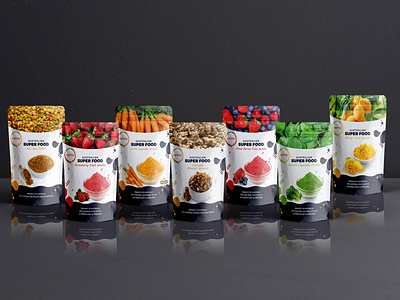This is a detailed image of seven sleek, white packets of various superfood powders, all neatly lined up on a glossy black surface against a dark gray background. Each packet is adorned with vibrant depictions of the superfoods contained within. From left to right, the products showcase a diverse array of nutritious ingredients: the first packet appears to feature lentils, followed by strawberries, then orange carrots. The fourth packet displays a bowl of walnuts, while the fifth shows a mix of berry powders with illustrated strawberries and blueberries. The sixth packet reveals a green leafy powder, likely spinach, and the packet at the far right depicts orange slices, suggesting mango. The white packets prominently feature the word "Superfood" amidst other less distinct lettering, capturing the essence of healthy, concentrated nutrition. Subtle shadows beneath each packet add depth to the composition, and the overall presentation emphasizes the variety and health benefits of these superfoods.